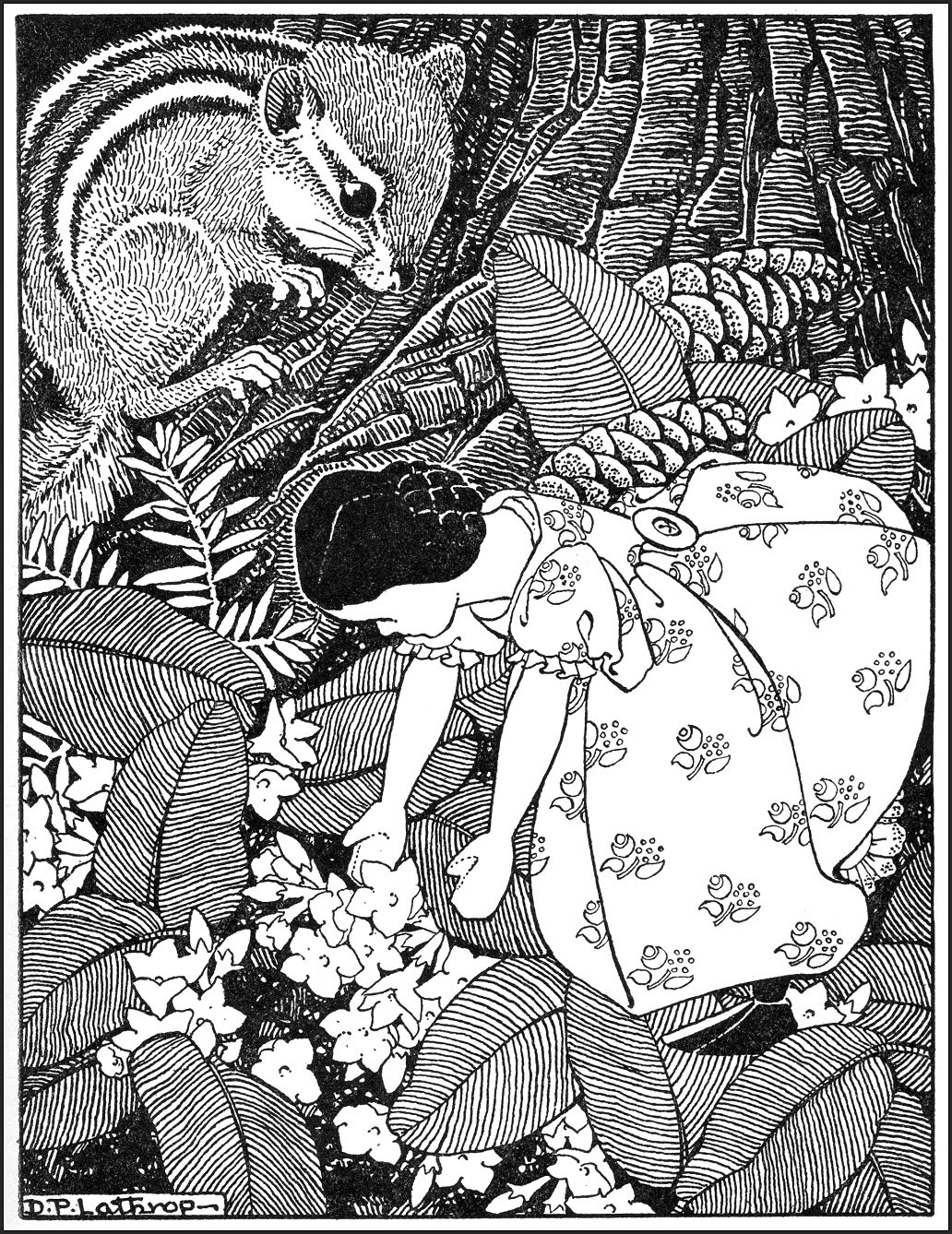This intricate black and white ink drawing depicts a forest scene where a little girl, resembling a doll, is central to the image. The girl, with black hair pulled back into a bun, is dressed in a flowery, puff-sleeved dress that billows out gracefully. She is bending down, her arms outstretched, reaching to pick a tiny white flower from among a dense array of meticulously line-drawn leaves and flowers on the forest floor. In her hand, she already holds a flower. The background features additional floral elements, twigs, and pine cones scattered across the forest floor. To the left of the girl, a large, curious squirrel—almost as big as the girl—is gazing down at her from the base of a massive tree trunk. The artist's signature, "D.P. Lanthrope," is inscribed at the bottom, adding a personal touch to this captivating portrayal of a serene woodland moment.